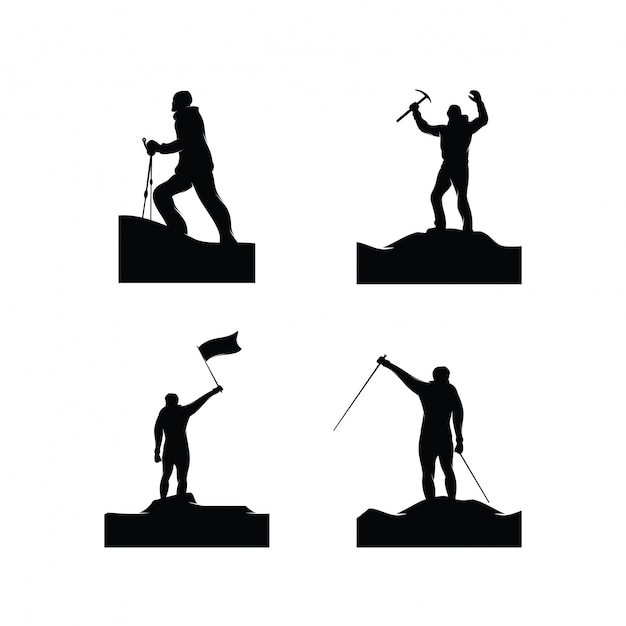This image consists of four black and white illustrations arranged in a two-by-two grid, each depicting a silhouette of a man engaged in various stages of a mountain climb. The top-left illustration shows a man hiking uphill with two walking sticks for support. The top-right image portrays the man standing triumphantly on a mound, raising a pickaxe above his head with both hands. In the bottom-left illustration, the man holds a flag aloft in one hand while standing on a summit, with the other hand rested by his side. The bottom-right image features the man standing with one hiking stick held upwards and the other down by his side. All images are black silhouettes against a white background, capturing a sense of progression and achievement through the climb. The man is consistently depicted wearing a beanie and gloves.